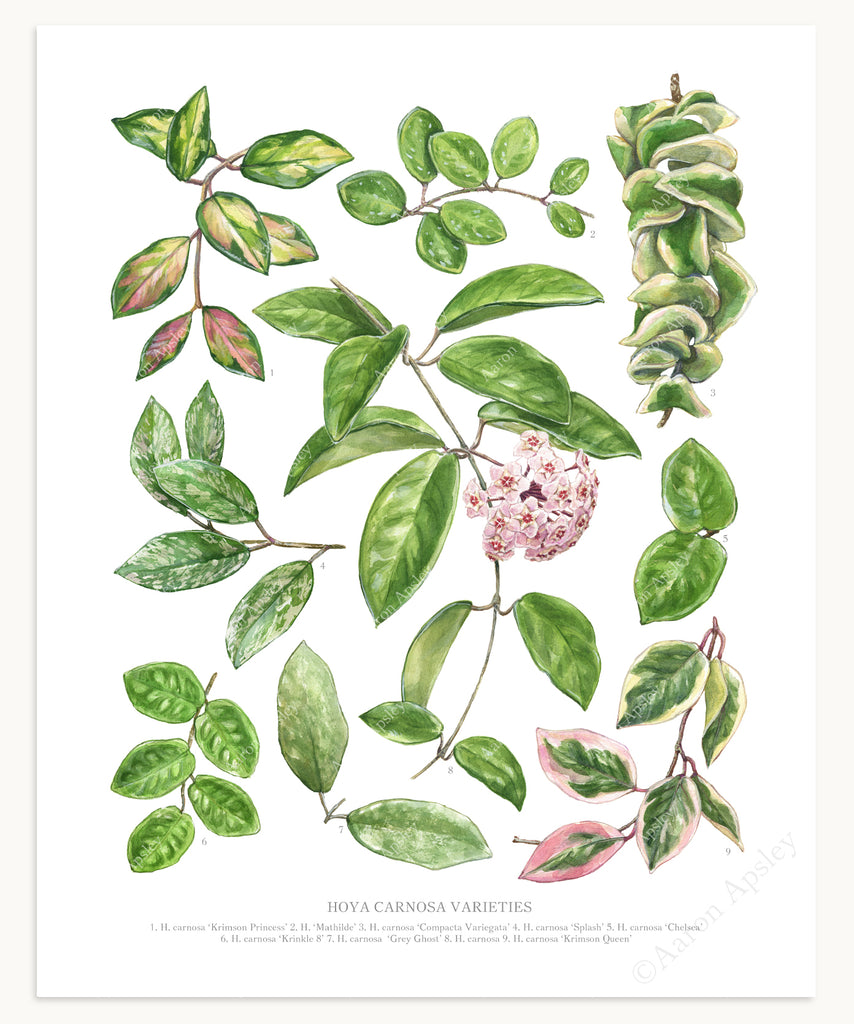The image is a finely detailed botanical illustration of Hoya Carnosa varieties, seemingly taken from a botany book or presented as professional artwork. Rendered on a clean, matte ivory background, it showcases nine distinct illustrations of the Hoya carnosa plant and its cultivars. At the center of the image is a thin green stem adorned with bright green, oval-shaped leaves interspersed with red-centered pink flowers in full bloom. Surrounding the central illustration are various leaf configurations, including some that are heart-shaped and others forming tight garlands. These leaves exhibit a mix of colors; some are purely green, while others display variegated patterns with patches of pink, white, or ivory. Beneath the main illustration, the text "Hoya Carnosa Varieties" is clearly printed, though additional smaller text beneath it remains too faint to read. A watermark of the artist's name, Aaron Apsley, is also present, reinforcing its authenticity as a piece of fine art. The Hoya carnosa, known for its tropical origins in Southeast Asia and popularity as a houseplant, is beautifully captured in this watercolor illustration.